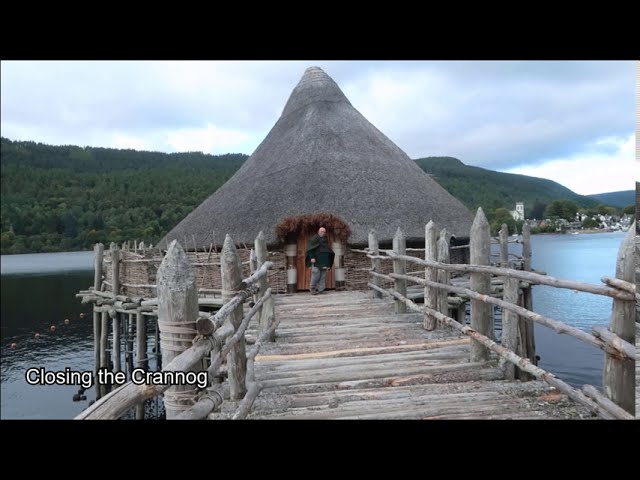The photograph, framed with black bars at the top and bottom, depicts a rustic scene taken during the daytime. The setting features a primitive wooden pier made from weathered gray logs tied together with thick ropes, extending over a calm body of water. The pier leads to a round structure with a large conical-shaped roof, identified as a crannog. The vertical pylons around the pier have sharpened, pointed ends, adding to the primitive aesthetic. Standing in front of the wooden door that serves as the entrance to the crannog is a bald man of Caucasian descent, dressed in a dark brown cloak and tunic over gray pants. The background reveals tree-covered hills and a small town on the right-hand side of the shoreline. Above the scene is a mostly cloudy sky with blue, gray, and purple clouds. There is also a line of buoys in the water on the left side. In white print with a black outline, located just over the bottom left corner of the pier, is the text, "Closing the Crannog."